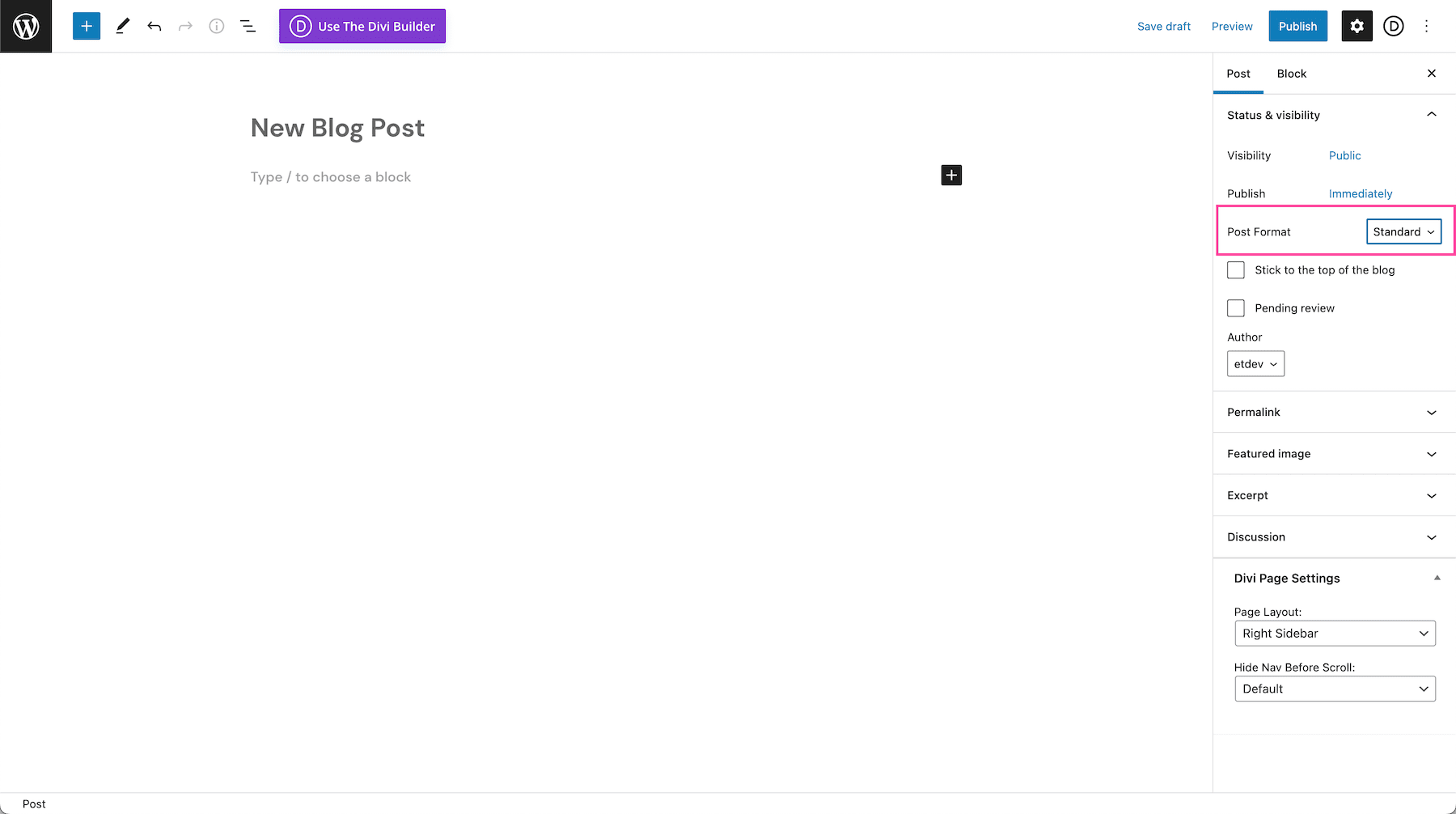The image showcases the interface of a WordPress webpage under the "Categories" section. At the top left corner, the iconic WordPress logo is visible alongside a plus sign, an edit button, and a back arrow. A prominent purple bar runs horizontally across the top of the screen, featuring a circular "D" icon and text that reads "Use the DB Builder."

Moving right along this top bar, there are options for "Save Draft," "Preview," "Publish," a black settings button, and another circular "D" icon. Below this bar, the main interface indicates the creation of a "New Blog Post." Here, users are prompted to "Type" and "Choose a block," but this area is currently blank.

On the right-hand sidebar, multiple sections are visible, including:

- Post or Block settings
- Status and Visibility: with visibility set to "Public" and the option to "Publish immediately."
- Post Format: set to "Standard"
- Additional options like "Stick to the top of the blog," "Pending Review," and author listed as "ELDEV"
- Other sections for "Permalink," "Featured Image," "Excerpt," "Discussion," and "DB Page Settings."

The page layout displays "Right Sidebar," with settings for "Hide Nav Before Scroll" defaulted. The image appears to capture the preparatory stages of drafting a blog post, with much white space indicating that content has yet to be added.